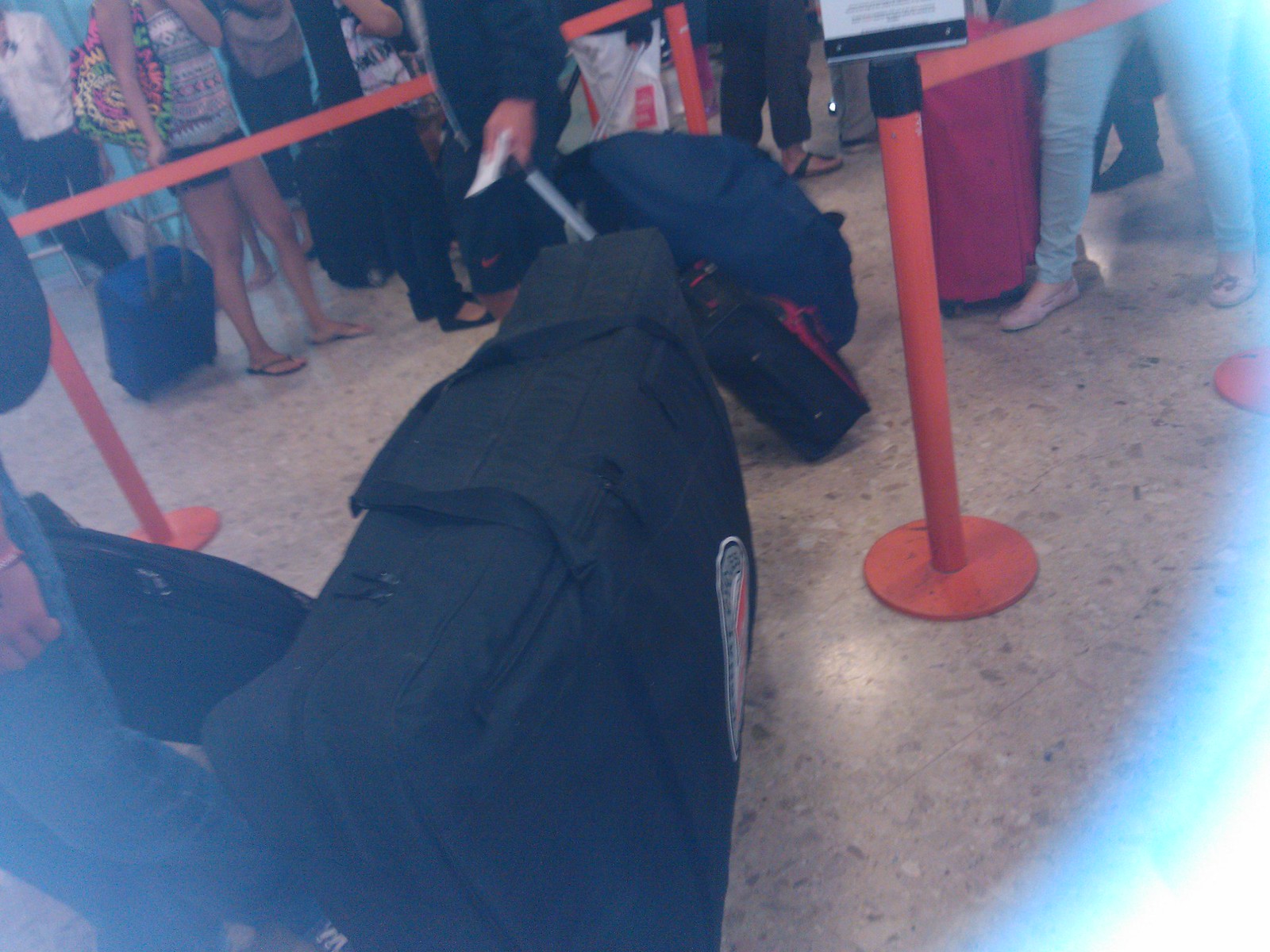In this image taken at an airport, a diverse group of travelers are standing in line, each with various types of luggage. The scene is primarily focused on the lower halves of people, showing a mix of legs and suitcases in different styles and colors. Notably, there is a woman in blue jeans with a large red cloth suitcase on her right. Nearby, a man in dark clothing is pulling a black suitcase topped with a large navy blue bag. Another noticeable feature is a very large black tote bag, stuffed to the brim, on the floor close to someone in light blue jeans. 

To the right, the legs of a girl in blue jeans are visible, and a distinctive hot pink suitcase sits beside her. One woman, dressed in shorts and sandals, stands with a navy blue pull suitcase and a colorful bag slung over her arm. Multiple people in varying outfits are scattered throughout the background, standing in line behind red stream barricades that form a zig-zag pattern to manage the queue. The floor is a beige-tan, spotted tile. The photo itself has some overexposure, particularly visible as circular glare marks at the top right and bottom corners of the image. No faces are visible, emphasizing the anonymity and bustle typical of a crowded airport scene.